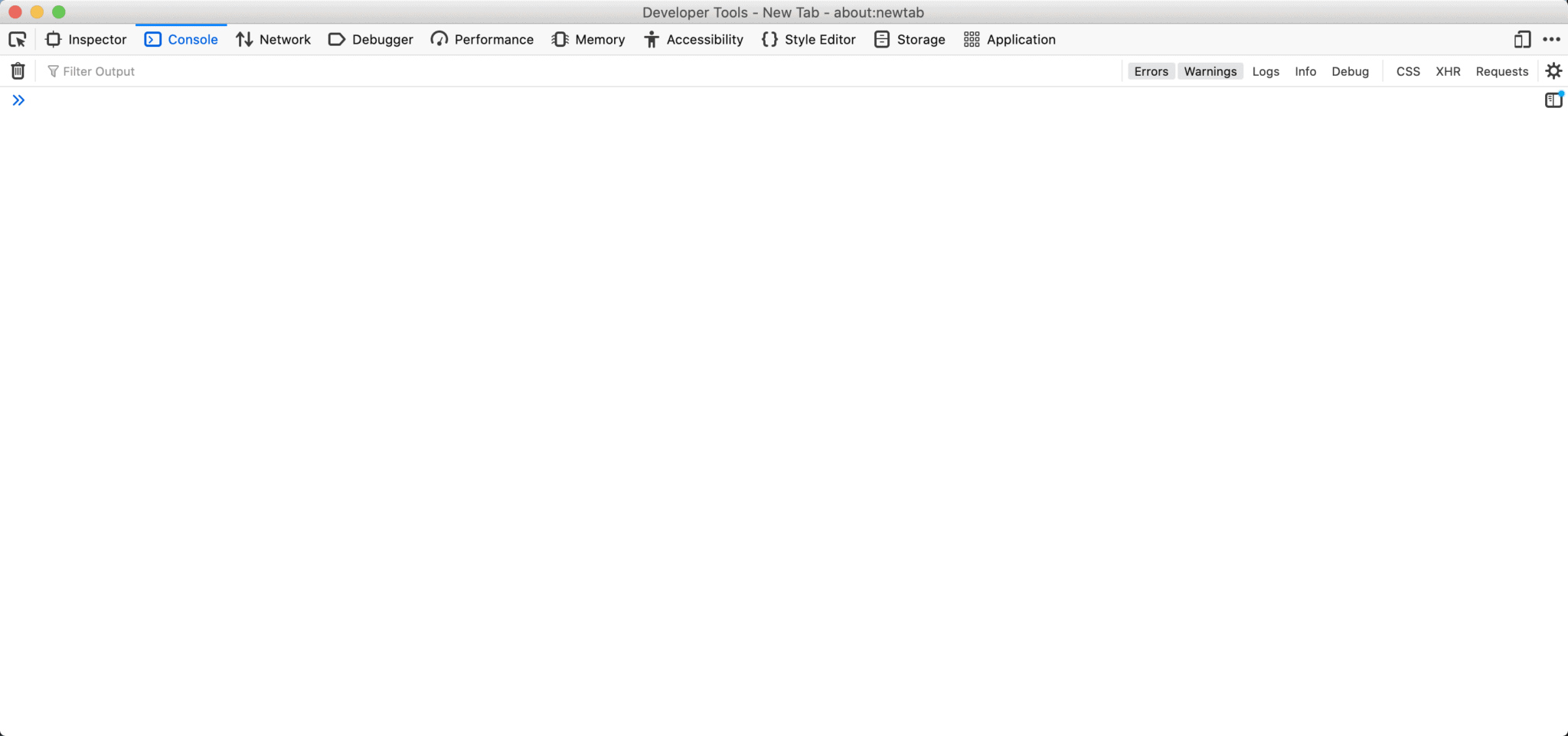This image showcases the Safari web browser interface on an Apple device. Prominently featured at the top-left corner are the standard macOS window control buttons: a red circle for closing the window, a yellow circle for minimizing it, and a green circle for maximizing or resizing. Directly beneath these controls lies the browser's tab bar, displaying several open tabs with options such as "Developer Tools," "New Tab," and "About."

The central area of the screen is occupied by the Developer Tools panel, segmented into multiple sections. These sections include:

- **Inspector:** A detailed DOM tree viewer for examining the HTML structure.
- **Console:** A console logging interface for executing JavaScript commands and viewing logging output.
- **Network:** A resource tracker for monitoring network traffic and debugging network requests.
- **Debugger:** A script debugger for setting breakpoints and stepping through code execution.
- **Performance:** Tools to analyze runtime performance and frame rates.
- **Memory:** Tools to investigate memory usage and detect memory leaks.
- **Accessibility:** Evaluation tools for improving web accessibility.
- **Style Editor:** Interface for editing CSS stylesheets live.
- **Storage:** Examination tools for local storage, session storage, and cookies.
- **Application:** Utility for inspecting various web application components, such as service workers and manifest files.

Below these tools is the "Filter Output" section, offering various options for refining what types of logs are displayed, including errors, warnings, logs, info messages, debug messages, CSS issues, XHR requests, and general network requests.

The bottom portion of the screen is mostly white space, likely reserved for dynamic output or more detailed content when interacting with the developer tools.